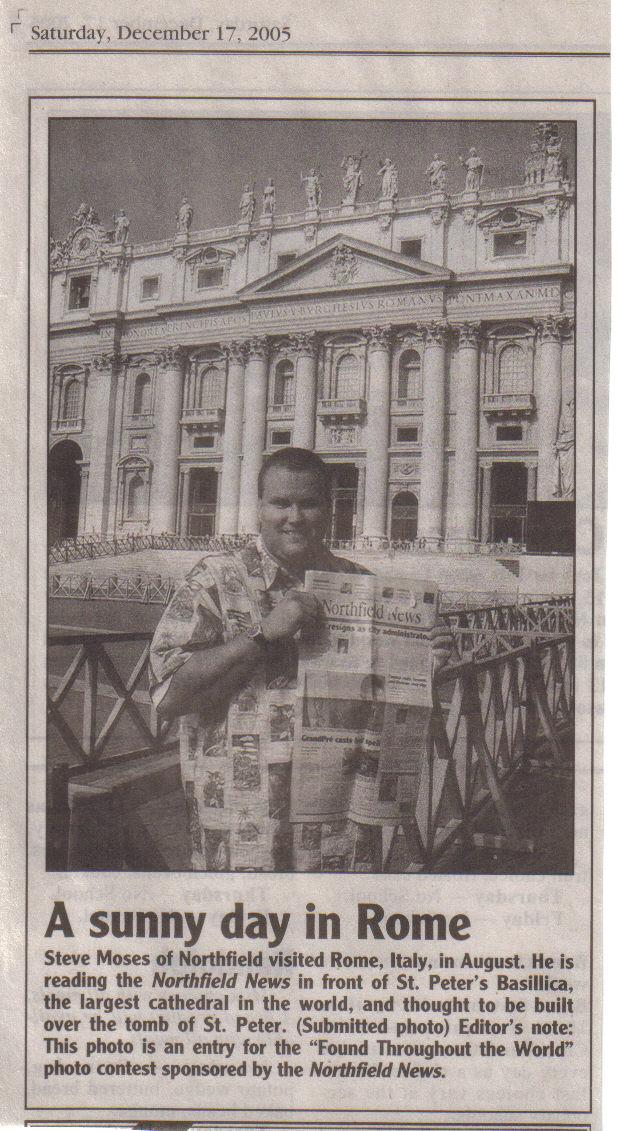The black-and-white image captures a newspaper clipping dated Saturday, December 17, 2005, at the top left. Below the date is a prominently featured photograph of a man named Steve Moses from Northfield. Steve, a larger white man, stands before the grand and historic St. Peter's Basilica in Rome, Italy. He is holding a copy of the "Northfield News" newspaper, with the vast, intricately detailed structure of St. Peter's Basilica visible behind him, complete with its traditional architectural elements and statues adorning the upper façade. The accompanying text beneath the photo highlights his visit in August, noting the significance of the basilica as the largest cathedral in the world, believed to be built over the tomb of St. Peter. The article further mentions that the photo, marked as a "submitted photo," is an entry for the "Found Throughout the World" photo contest organized by the Northfield News.